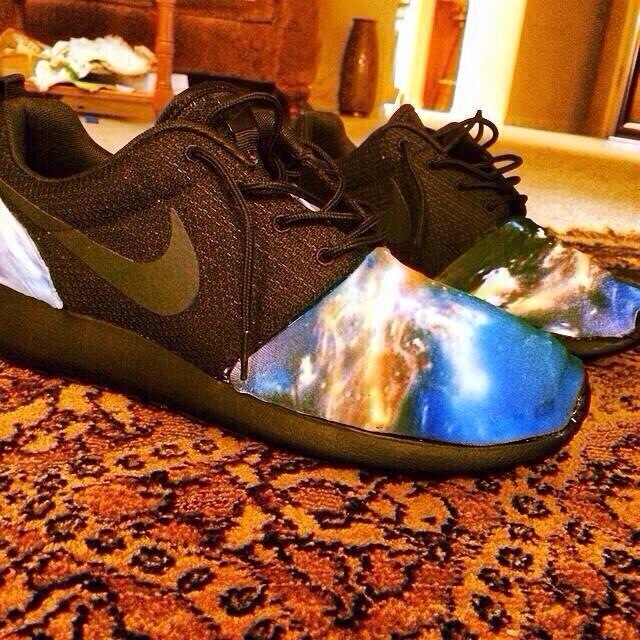The image depicts a detailed, full-color indoor scene, primarily focused on a pair of Nike tennis shoes. The shoes are prominently centered on a patterned carpet with a mix of yellow, black, brownish-orange, and red designs. The shoes themselves are predominantly brown with black features, including black shoelaces and a Nike swoosh, while the toe box and back heel are adorned with a spacey, multicolored design that shimmers like silver. Surrounding the shoes, the background reveals parts of a living space: a section of a couch, a wooden table with some garbage underneath, and a brown wooden vase. The scene, illuminated by natural daylight streaming in, suggests it’s taken in someone's house. The detailed carpet, which may actually be a distinct rug, transitions to a lighter-colored floor at the edges, contributing to the indoor ambiance.